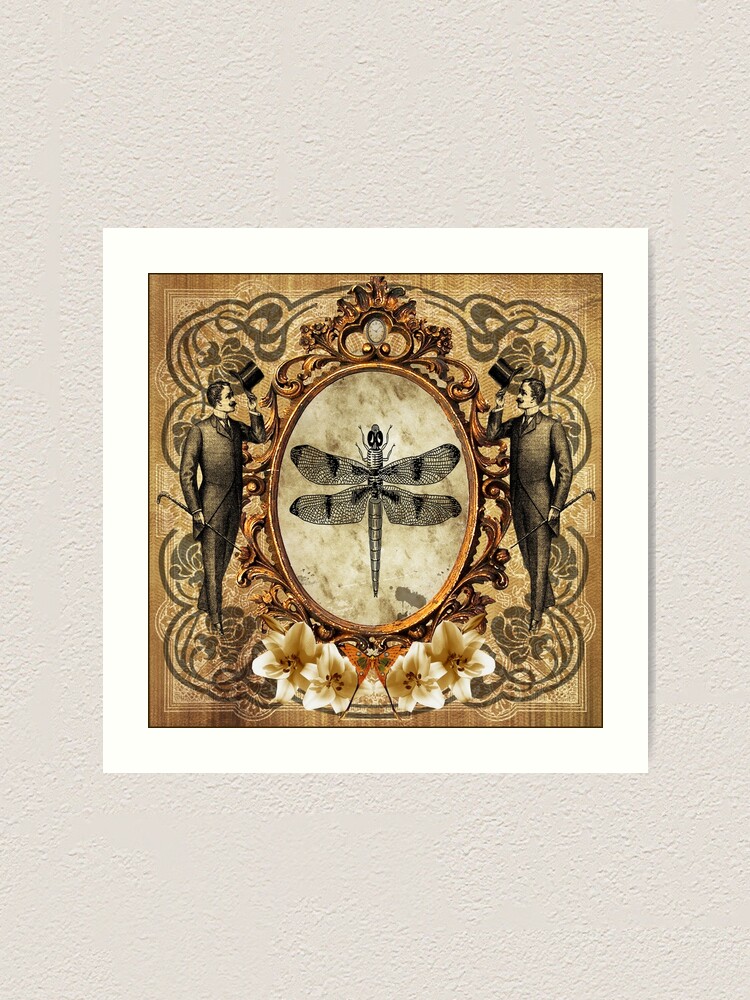The image portrays an intricate drawing of a dragonfly set within an oval frame that exudes a vintage turn-of-the-century charm. This central oval, which showcases the dragonfly in meticulous detail, is edged with a scrawled golden or bronze ornate border. The dragonfly, rendered in black ink with clear wings adorned with black dots and dashes, has a long body and a distinguishable head. Notably, only four of its legs are visible, likely obscured by the wings.

Flanking the dragonfly are identical gentlemen, each tipping a top hat with one hand while holding a cane in the other, suggesting a gesture of polite greeting. These figures, dressed in dark suits, provide a symmetrical balance to the composition, as they mirror each other on either side of the dragonfly.

Beneath this central vignette, the composition is enhanced by an arrangement of flowers and a small orange butterfly. The background of this detailed scene is a rich brown, which fades into a white border. The entire picture is set against an off-white, greyish stucco-like background, adding to the aged and classic aesthetic of the artwork.